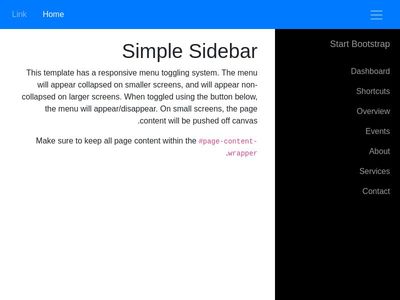The image depicts a user interface with several distinct elements. At the top of the interface, there is a prominent long blue bar. On the left side of this bar, the word "Link" appears, followed by the word "Home" in bold white text. Towards the far right side of the bar, there are three horizontal white lines.

Below these horizontal lines is a long black box, which contains a list of menu items starting from the top: "Start Bootstrap," "Dashboard," "Shortcuts," "Overview," "Events," "About," "Services," and "Contact." On the left side of the screen, the words "Simple Sidebar" are written, with each word capitalized.

Underneath these words, there is a paragraph that explains the functionality of the template's responsive menu toggling system. The text reads: "This template has a responsive menu toggling system. The menu will appear collapsed on smaller screens and will appear non-collapsed on larger screens. When toggled using the button below, the menu will appear/disappear. On small screens, the page content will be pushed off canvas."

Further below this explanatory text, there is an advisory note: "Make sure to keep all page content within the 'page-content' area." The phrase "page-content" is highlighted in pink text. At the bottom, the letters "APPR" are displayed prominently.